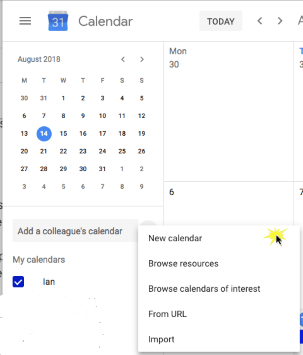A screenshot of a typical online calendar page for August 2018 is displayed. In the top left-hand corner, there are three horizontal lines, serving as the main menu icon. Adjacent to the menu icon, a blue box features the number "31" in white font, signifying the site’s primary calendar feature. Directly next to it, the word "Calendar" is written in black font.

Below the header, a navigation bar offers various calendar view options such as "Today," which is highlighted at the moment, as well as buttons to move forward, backward, or view the entire month. The main section displays the monthly view of the August 2018 calendar. Each day of the week is indicated by its initial letter, with the corresponding dates listed beneath them in columns. The date "14," representing Tuesday, August 14th, 2018, is distinctly highlighted, indicating a focus on that particular day for whatever event or information is being sought.